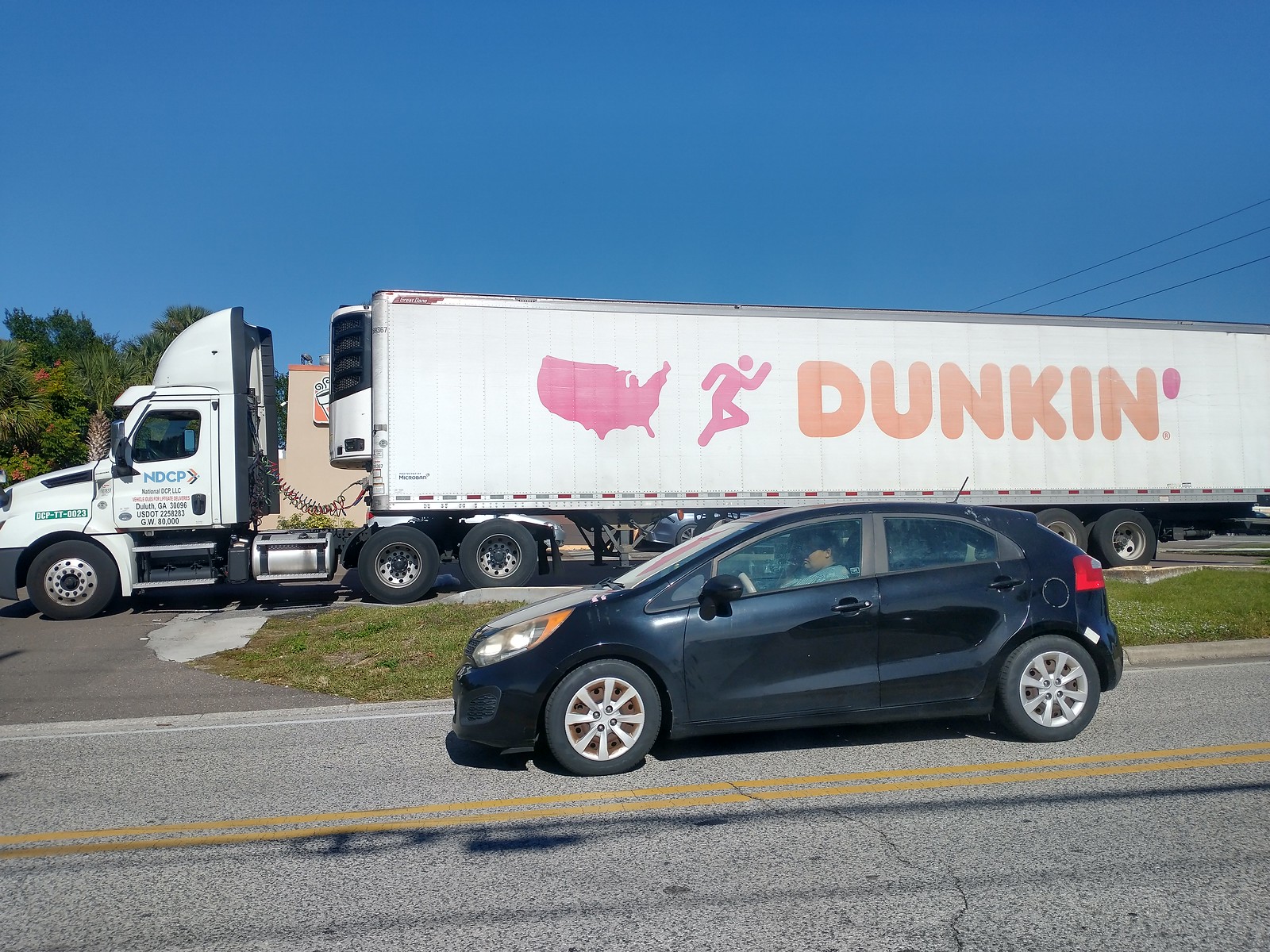The image is a landscape-oriented photograph taken outdoors on a highway. Dominating the foreground, a blue car is positioned along a yellow divider on a two-lane road, creating the impression it's either in motion or momentarily halted in the middle of the highway. Adjacent to this scene, on an access road beyond the median, a large white semi-truck is visible. The truck is branded with Dunkin' Donuts imagery, featuring a pink outline of the United States, a pink icon of a person running, and the word 'Dunkin'' in coral, with pink apostrophes. Behind the truck, a warehouse is partially visible, nestled among some trees. The scene is crowned by a clear blue sky, adding to the expansive and open-air feel of the highway setting.